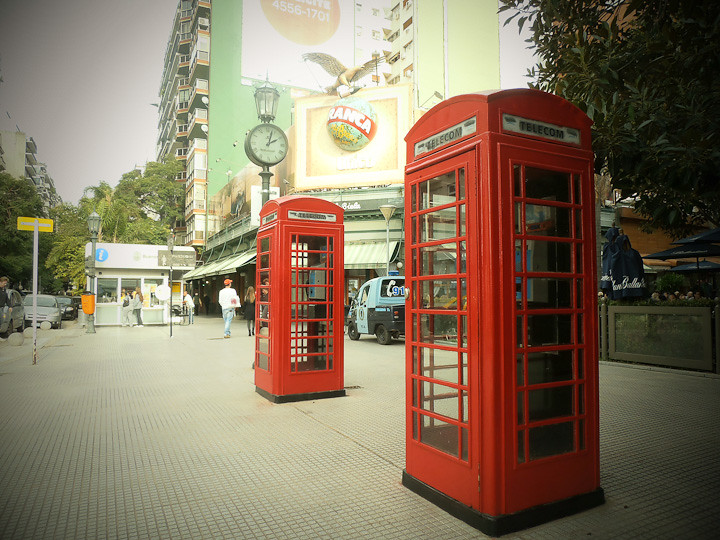The image is a colour photograph taken outdoors on a street that features two iconic red telephone booths, reminiscent of traditional London-style phone boxes with glass panels arranged horizontally within them. These phone booths are positioned prominently in the right foreground. The street itself is paved with tiny square tiles, leading the eye toward the background where people can be seen milling about. To the right, a large, green apartment building dominates the scene, with distinctive bay-type balcony windows lining the left side of its façade, receding into the distance.

The sky above is quite grey and slightly overcast, adding a muted tone to the urban landscape. Along the left edge of the image, vehicles are parked along the street, extending into the distance. In the upper right corner, a green tree is visible, and below it, a barrier suggests the presence of a restaurant, evidenced by the nearby folded blue awning tents. Additionally, a small light blue and black vehicle, possibly a parking meter truck, is noticeable with a partial phone number (9-1) on its back window.

Further details include a clock affixed to a tall post, showing a time slightly past 2 p.m. in Roman numerals, with a lamp perched above it. A billboard or sign near the apartment building displays the word "Blanca," and a globe with an eagle holding a champagne bottle can be seen atop the building, adding unique visual elements to the lively street scene.